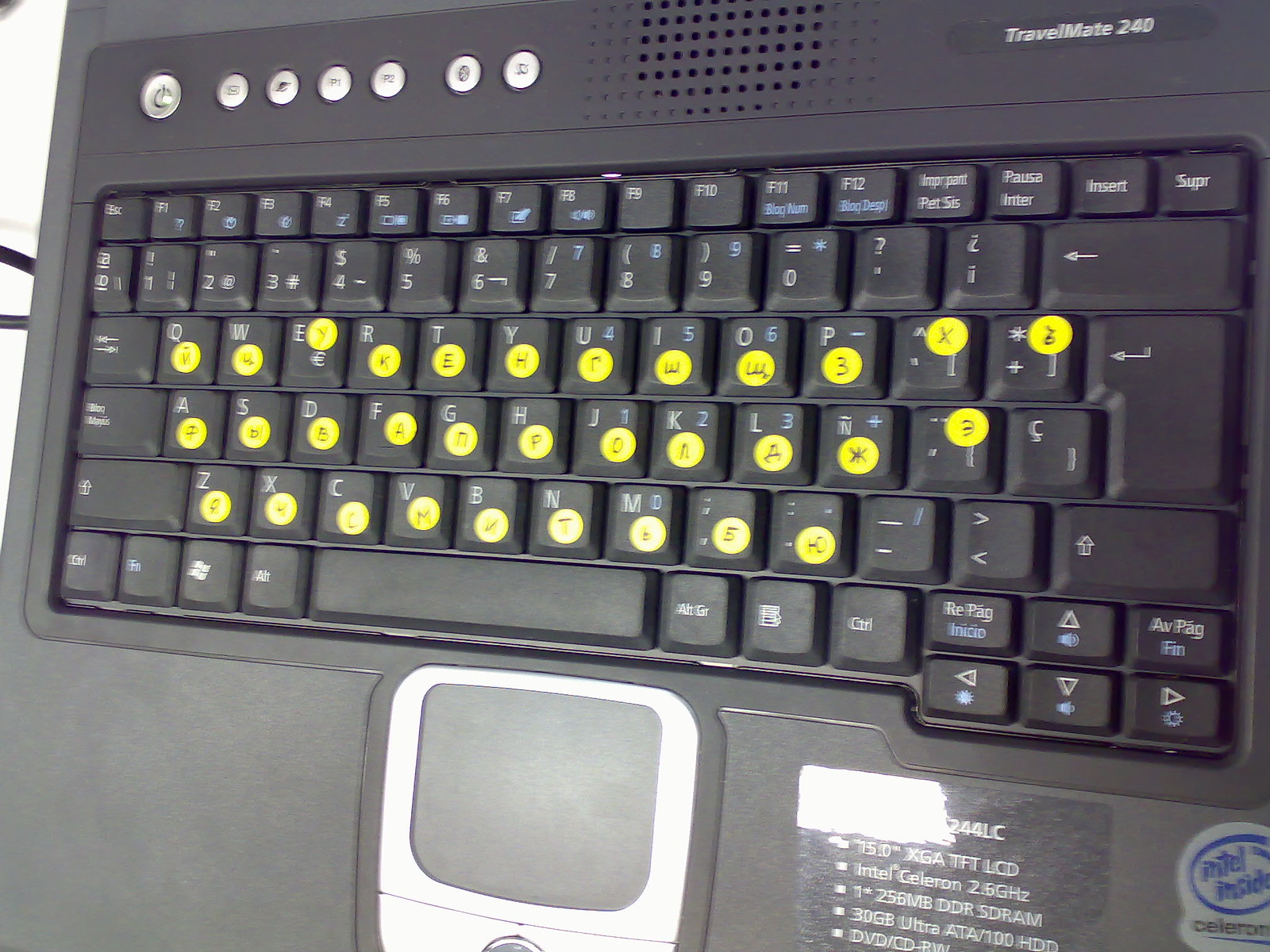The image depicts a blurry close-up of a black laptop keyboard, characterized by its white lettering and blue symbols. The keyboard is cluttered with several yellow circular stickers, each displaying alternative letters and symbols in black text. For instance, the Y key is labeled as H. The bottom right of the image reveals a label confirming an Intel Inside Celeron processor and additional specifications, including 256 megabytes of memory and a 30 GB Ultra ATA/100 HDD. This amateurish photograph, while unclear, showcases the detailed specifications and unique labellings of the laptop, which might suggest that it is equipped with a custom or conversion keyboard.